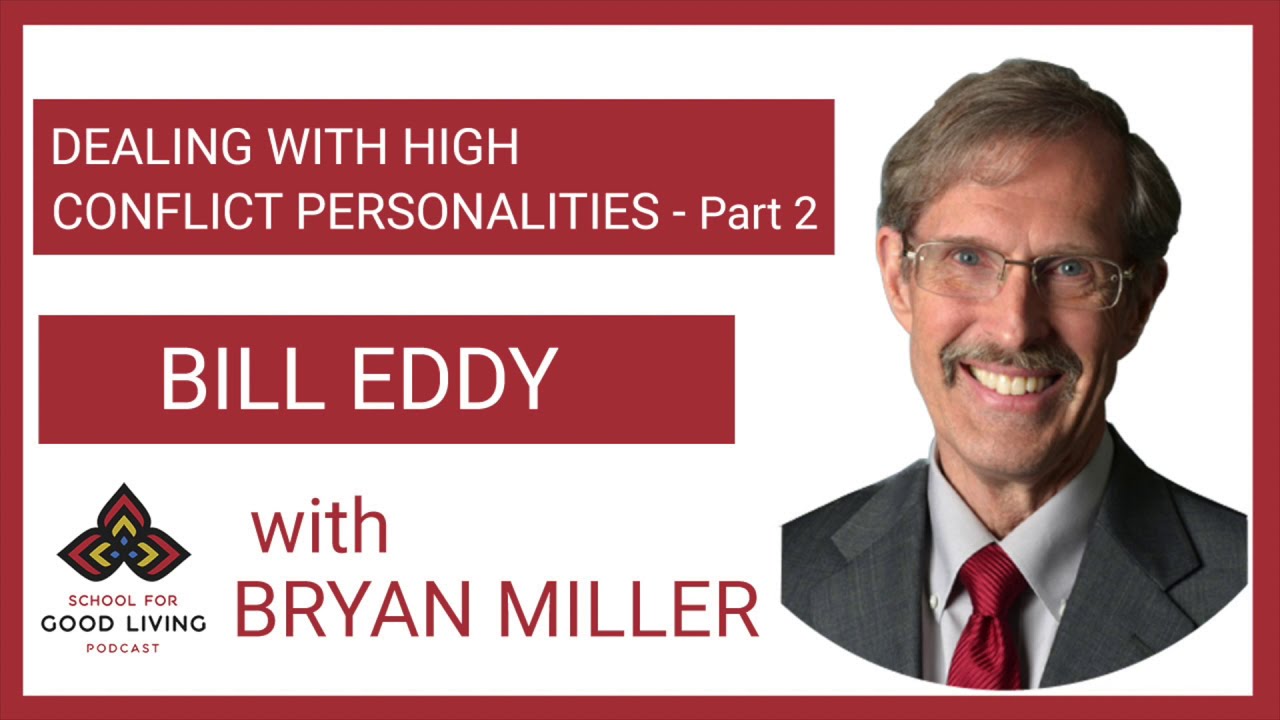The image appears to be a promotional advertisement for a podcast episode titled "Dealing with High Conflict Personalities - Part 2." The design features a dark red or maroon border, with a white background and red accents throughout. At the top left, within a red rectangular highlight with white letters, is the title of the episode. Below this, a smaller red rectangle with white text reads "Bill Eddy." 

Further down in the white background, also in red letters, it says "With Brian Miller." On the left side, there's the "School for Good Living Podcast" logo, which features a red, yellow, and blue three-leaf emblem. On the right side, there is a photograph of a smiling middle-aged man, likely in his early to mid-50s. He is depicted with thinning, light brown hair, blue eyes, and a handlebar mustache. He wears glasses and is dressed in a dark gray suit, a lighter gray dress shirt, and a dark red striped tie. The overall impression is that the image is promoting an engaging podcast episode featuring Brian Miller and guest speaker Bill Eddy, focused on navigating high-conflict personalities.